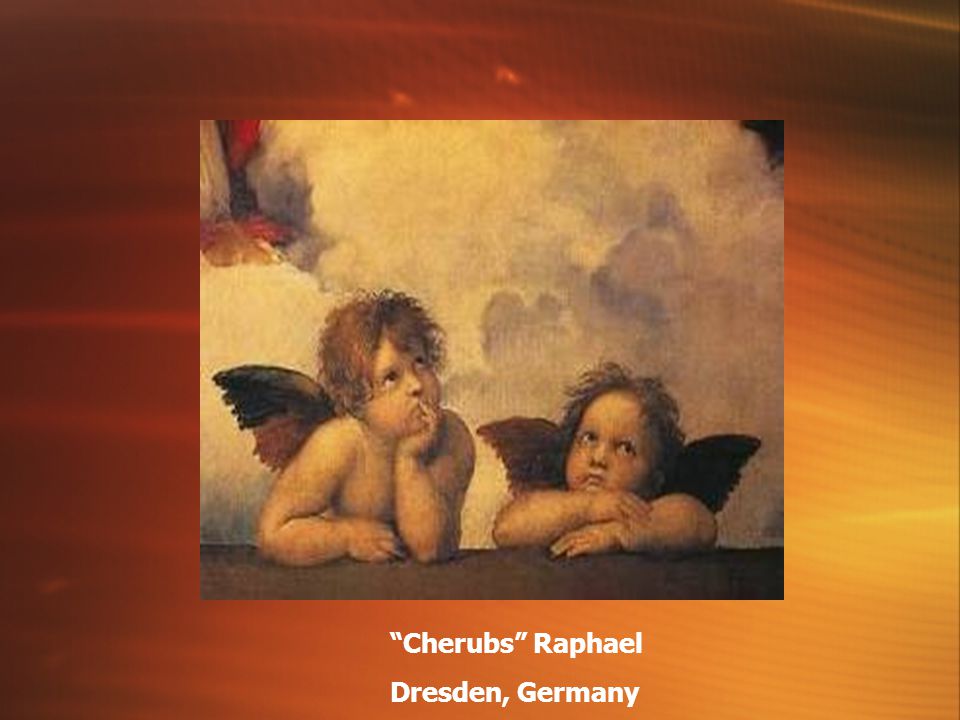The image is a slightly blurry photograph of a painting depicting two cherubic baby angels with small, bird-like wings in black and red hues. Both cherubs, with their curly brown hair, are gazing upward. The cherub on the left has its left hand touching its chin, while the other hand rests on a brown surface, which appears to be a table. The other cherub is also leaning on the table, with its arms folded. Fluffy white clouds are positioned behind them, suggesting a heavenly setting. The background of the painting blends light tan, yellow, orange, and red colors. Additionally, at the bottom of the image, text reads "Cherubs," "Raphael," and "Dresden, Germany" in white.